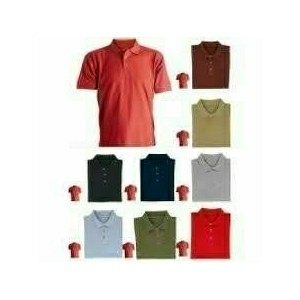This image is a product photo showcasing a variety of men's short-sleeved polo shirts arranged in a neat grid. The upper left-hand corner features a large, unfolded red polo shirt displayed as though being worn on a mannequin or model. Surrounding this main shirt are eight smaller folded polos, each accompanied by a tiny icon of the red polo, reflecting the larger one. These smaller shirts are only partially visible, showing just the collars and two buttons. From left to right, the colors of these polos are organized in three columns. The left column consists of orange, light blue, and a pale blue. The middle column features brown at the top, dark blue, and forest green. The right column contains lime green, an off-white color, and fire engine red at the bottom. Each shirt has three buttons running from the collar to the upper chest area, contributing to the detailed and organized display.